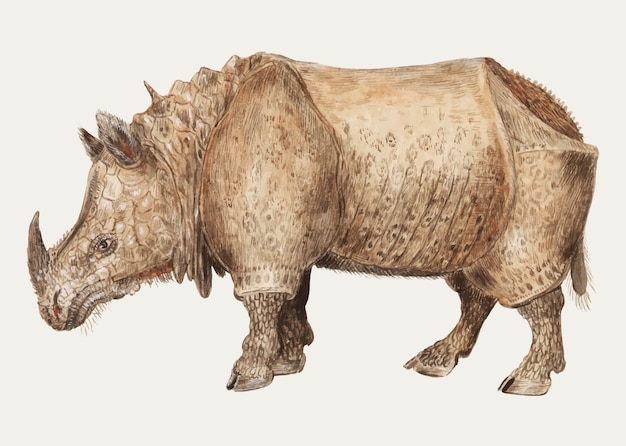The image depicts a large, one-horned rhinoceros standing on all four legs with a no-nonsense expression on its face. This rhinoceros, colored in golden-brown hues with tinges of light golden brown, appears to be wearing an elaborate set of armor that extends over its body and the top part of its legs, leaving its hooves uncovered. The armor-like skin features intricate details, including marks on its sides and belly, as well as scale patterns on its feet. The head of the rhinoceros also seems armored, and there is a noticeable horn at the top of its nose. The depiction is highly detailed and realistic, with blood visible coming from its nose, enhancing the dramatic effect. The artwork, which could either be a painting or digital art, is set against a light grey background.